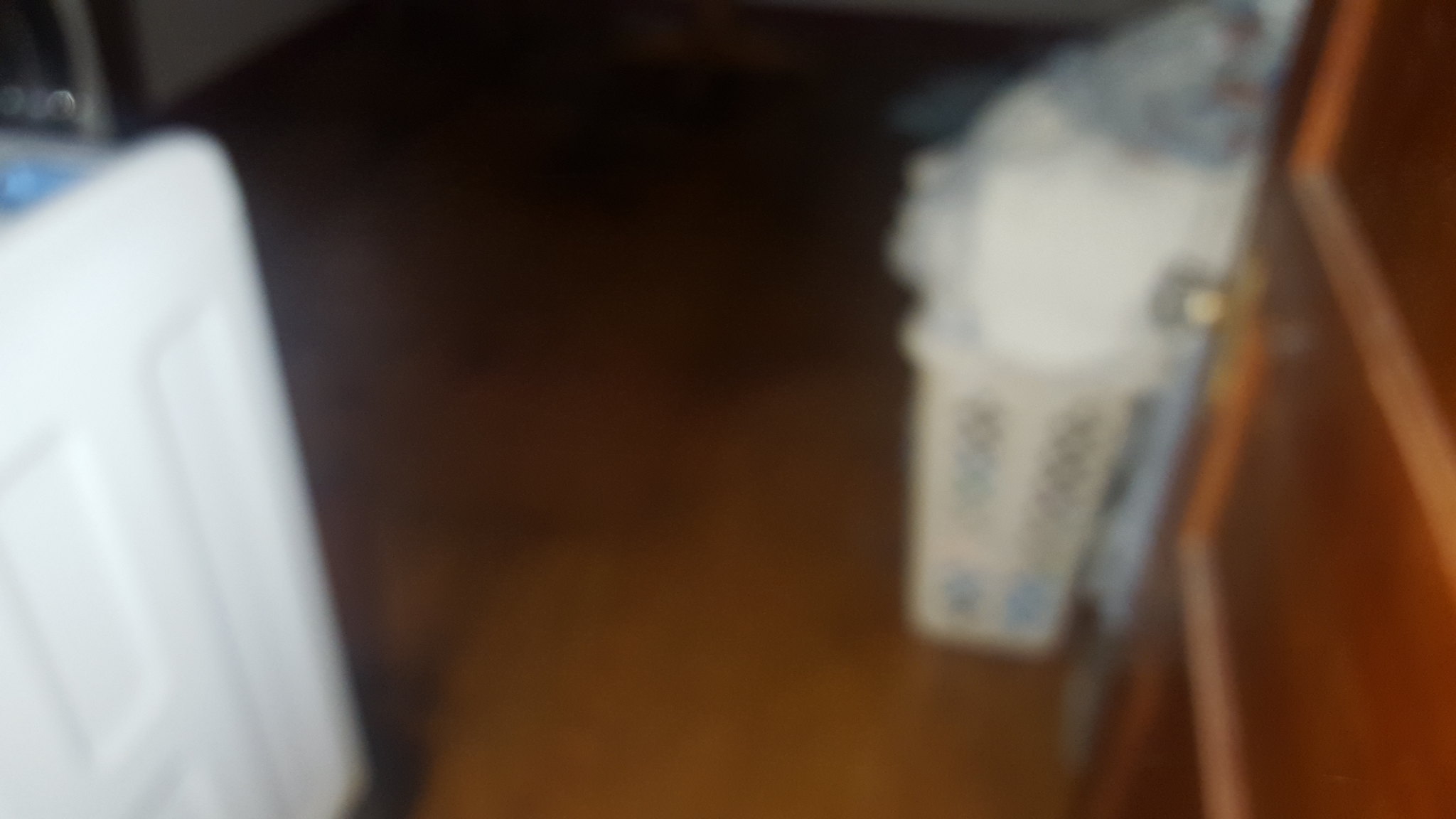A very blurry color photograph capturing the inside of a home. On the right side of the image, a dark brown door with a brass handle is slightly ajar, revealing a cluttered room beyond. Near the door, a white laundry hamper filled to overflowing with linens and blankets dominates the foreground. The linens appear to include white and gray sheets that spill over the side. On the left side of the room, a white object that might be a sink is visible, though it's hard to discern due to the blurriness. The upper left corner of the image is dark, almost black, possibly obscured by poor lighting or shadows. The flooring appears to be a false hardwood, although its features are indistinct. The small room also includes a partial view of another doorway or closet in the upper left section, adding to the sense of clutter and narrow space.